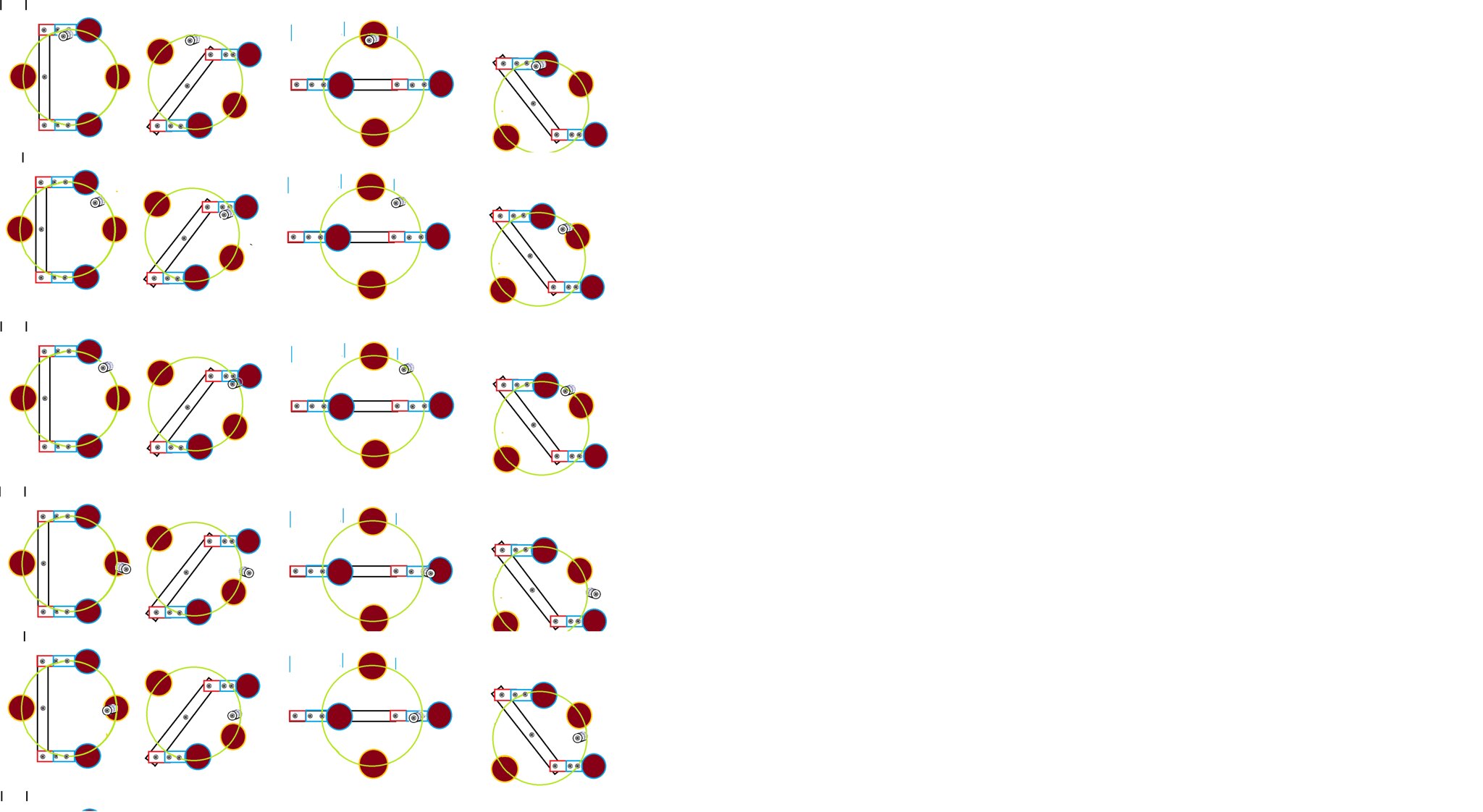The image depicts a detailed diagram positioned mostly on the left-hand side of the frame, leaving a significant white space on the right. The diagram displays a sequence of four distinct yet similar shapes arranged in rows, each representing a different stage of transformation within a frame structure. 

Starting from the left, the first shape resembles the letter "D," featuring prominent red circles at its endpoints and along its vertical sides. The second shape shows a frame shifting forward, causing the red circles to move accordingly. In the third column, the shape aligns into a straight horizontal line, with red dots positioned at the top, bottom, left, and right, indicating a balanced alignment of the frame. The final shape illustrates the frame tilting backward, maintaining the red endpoints and red circles along its length. All shapes are encompassed within a yellow circle that connects and encircles each segment, unifying the entire composition.